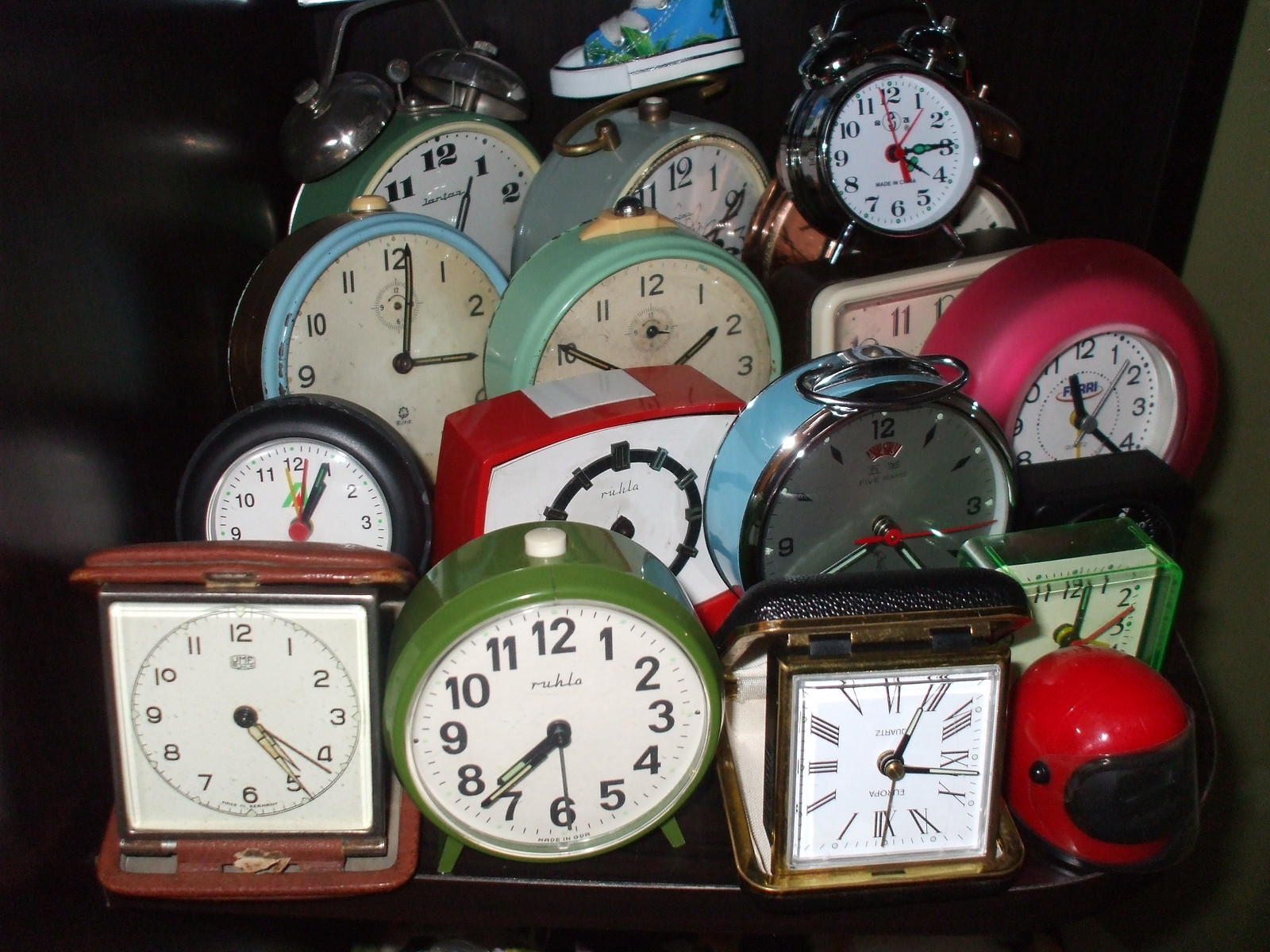The photograph captures a vibrant arrangement of 14 vintage-style analog clocks, stacked in a four-by-four grid on a small table. These clocks come in an array of colors; notable hues include light green, turquoise, gray, black, white, pink, light blue, red, brown, forest green, black with gold trim, and a unique transparent green. Most of the clocks are round, though there are a few with square faces designed as compact travel clocks that fold into a case. Some clocks are adorned with classic alarm bells on top, and a couple feature Roman numerals. In the lower right corner lies a miniature red motorcycle helmet, and atop one of the clocks sits a tiny baby shoe characterized by its blue, green, and white colors.